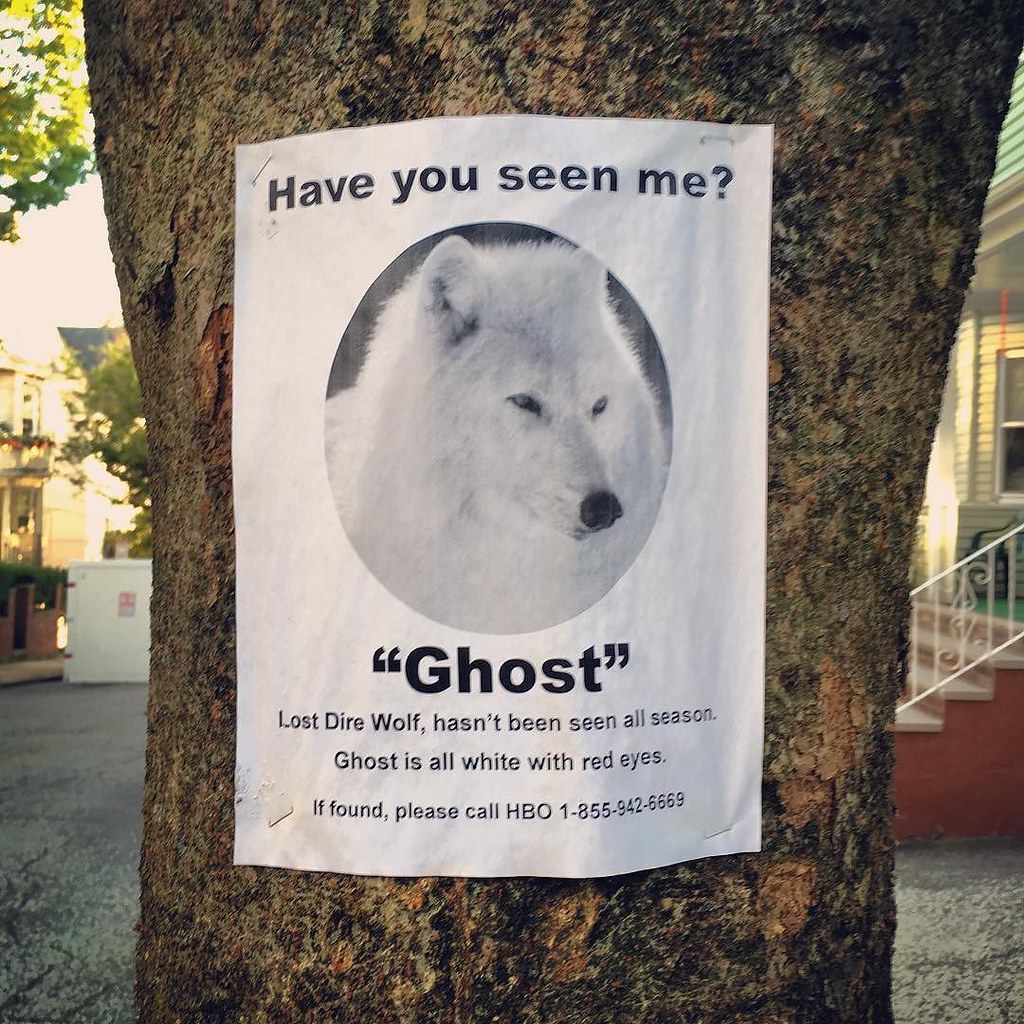The image depicts a missing poster for a dog stapled to a large, dark brown tree trunk. The poster is a white sheet with bold, black letters at the top asking, "Have you seen me?". The featured animal is a large, white dog resembling a collie or possibly a wolf. The name "Ghost" is highlighted in thick, black letters with quotes. The text underneath reads, "Lost dire wolf, hasn't been seen all season. Ghost is all white with red eyes. If found, please call HBO at 1-855-942-6669." The background includes a glimpse of a white house with a stairwell, red steps, and a window on the right, as well as green trees and an asphalt driveway on the left. The prominent colors in the scene are brown from the tree trunk, yellow, reddish-orange at the base of the steps, white from the poster and the house, and green from the trees and leaves. There are no people visible in the photograph.